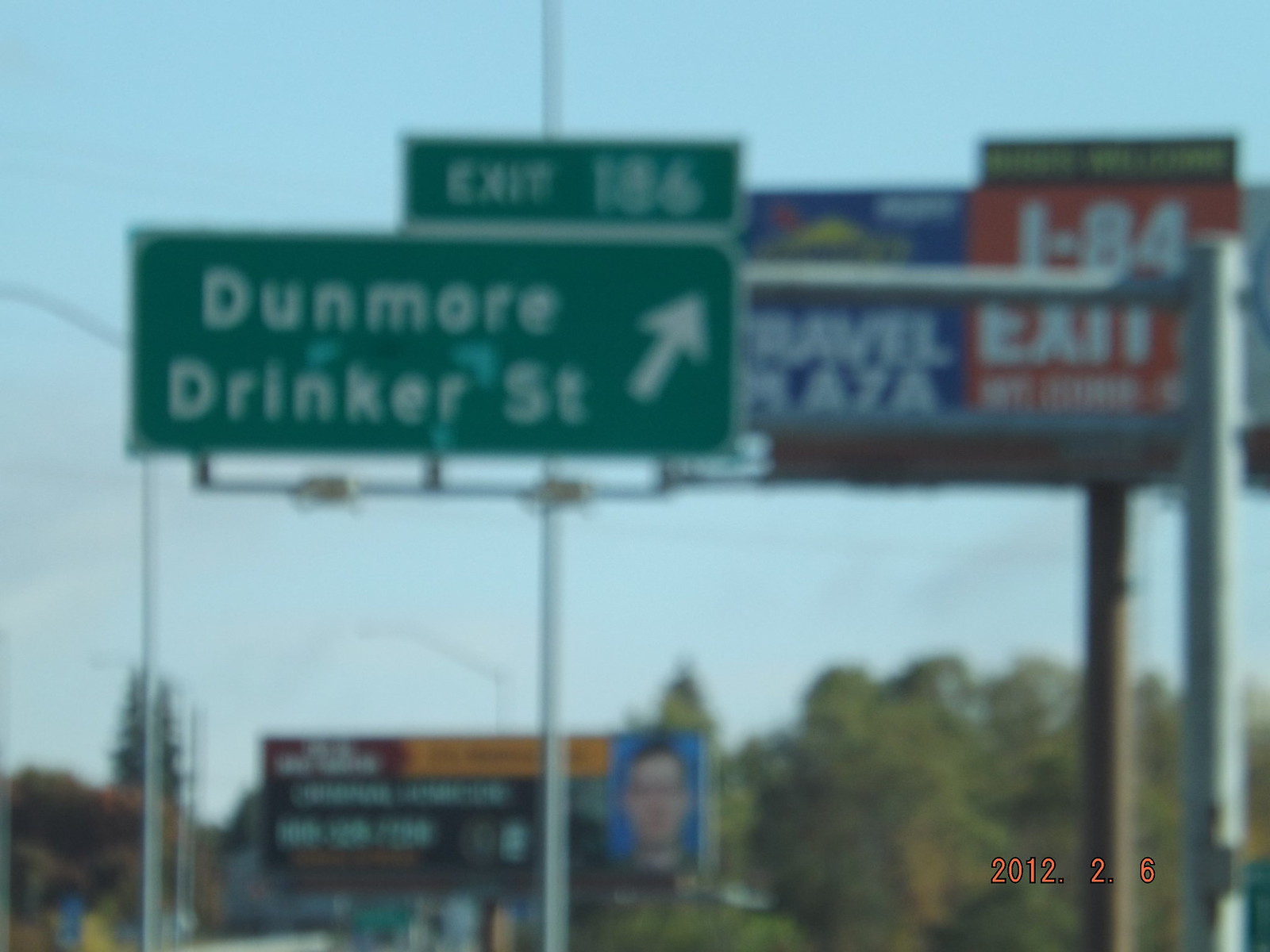This photograph, taken on February 6, 2012, captures a slightly blurry green road sign which is clearly the main focus of the image. The sign, part of a highway or freeway system, directs drivers towards Exit 186 for Dunmore Drinker Street, with bold white text and an arrow indicating the exit direction. The sign is mounted on a sturdy post connected to the roadside. In the background to the right of the sign, a billboard is visible, accompanied by another billboard further below in the mid-distance. The backdrop features a blur of green trees, adding a touch of nature to the road scene. The date "2012.2.6" is visible in the bottom right corner of the photograph.